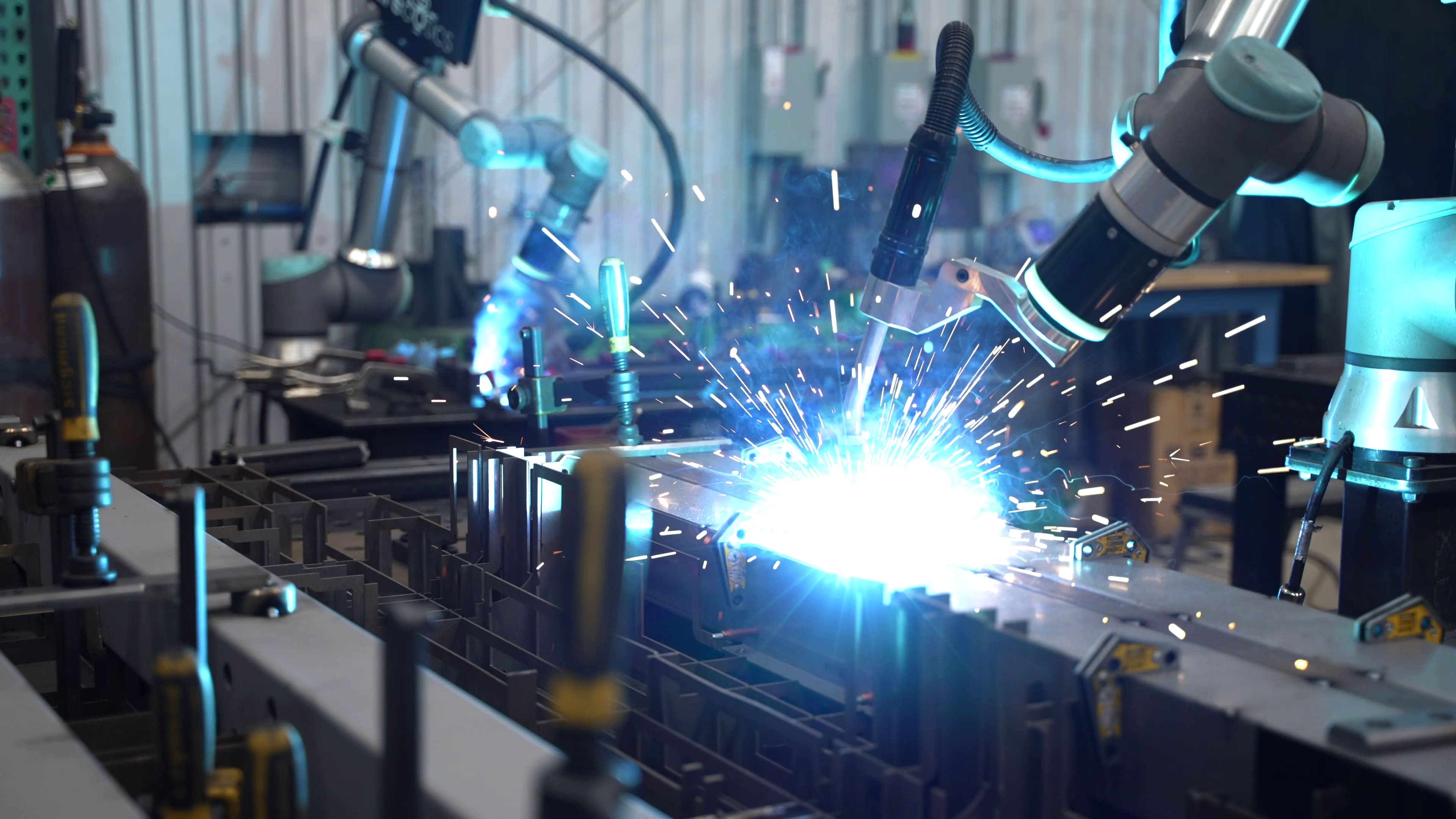The image depicts an industrial setting focused on advanced welding machinery, likely within a factory environment. Central to the image are robotic arms equipped with computerized controls, engaging in a welding operation on a piece of metal situated on a large work table. The welding process emits intense white light with a distinctive bluish tint at the edges, illuminating blue sparks. The robotic arms themselves are composed of metal poles with black tops, and incorporate black, silver, and gray components, along with small blue plastic pieces. To the left, another identical welding machine can be discerned, though its light appears dimmer due to its distance. The background reveals a light gray metallic wall with vertical lines and various attachments, reinforcing the industrial ambiance. Notably, there are no human workers visible, indicating the welding process is fully automated.